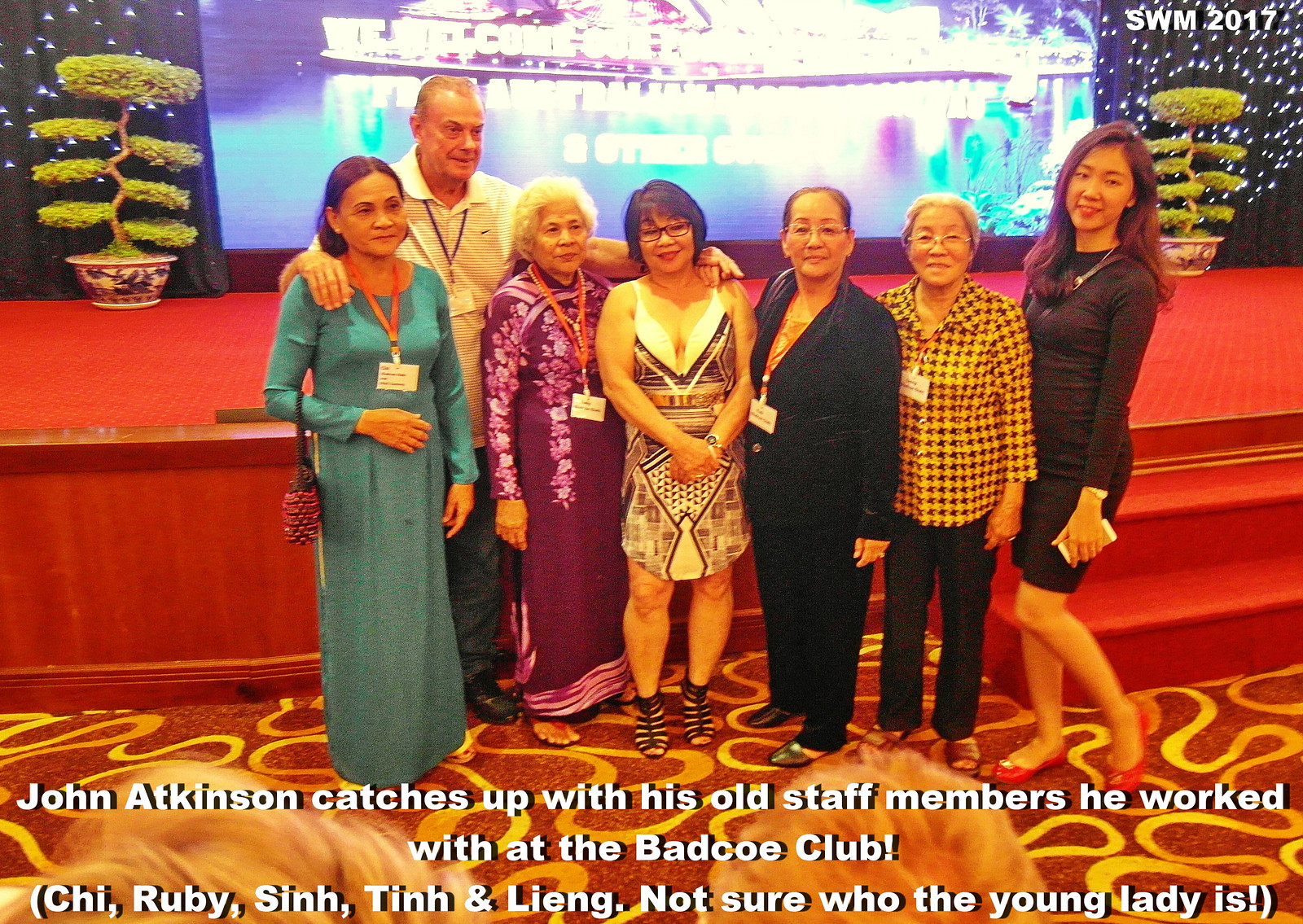The photograph captures a nostalgic reunion featuring a group of seven individuals standing in front of a red stage. The stage is adorned with a large, unreadable screen and flanked by two potted topiary trees. In the group, there are five older women and one younger woman positioned to the right, all wearing dresses or dressy clothes. They are joined by a man with long arms standing behind them, with his arms around three of the women. Most of the individuals are wearing lanyards with name tags. The setting suggests an event, possibly in a hotel lobby in Asia or Southeast Asia. A caption at the bottom reads: "John Atkinson catches up with his old staff members he worked with at the Batco Club. Chi, Ruby, Sin, Tin, and Woon; not sure who the young lady is."